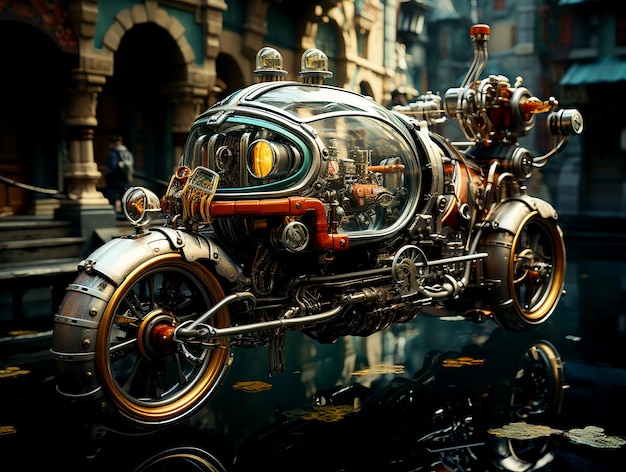This is a highly detailed 3D rendering of a futuristic, steampunk-inspired motorcycle, primarily chrome and gold in color, festooned with chrome pipes and gears. The two large wheels, featuring orange rims, black spokes, and metal strips or sheets of armor, are nearly fully enclosed by housings. The housing and overall structure exude a steampunk aesthetic, with numerous visible bolts, gears, and pistons—some in orange and silver—adding to its complex design.

A clear plexiglass capsule replaces the traditional seat area, encompassing the engine, gears, and other mechanical components. This capsule doubles as the headlight housing and features additional rotating dome lights and orange cylinders with an unusual substance emanating from them. The motorcycle sits on a reflective, glass-like road, dotted with a few leaves that enhance its shiny surface.

The background reveals a grand, arched building with cyan and gray bricks, through which a blurred man in a black cap, white shirt, and black pants is walking. The scene exudes a universally futuristic feel, unmatched by any conventional motorcycle seen on the road, making it a true visual marvel of imaginative engineering.